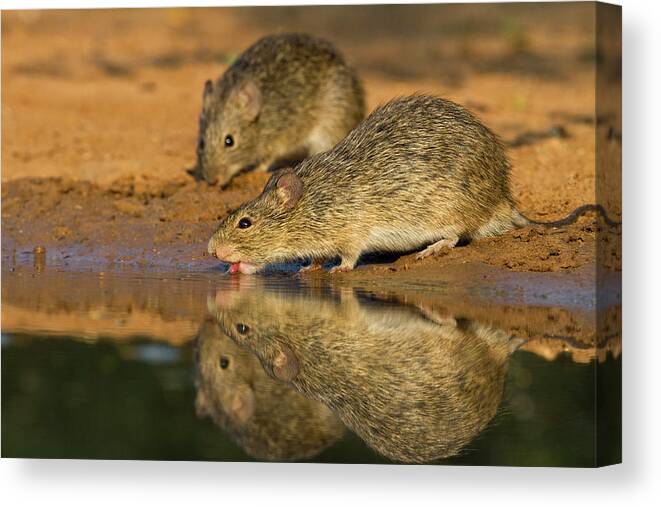In a stunning high-definition nature photograph, two large rats are captured drinking from a clear pool of water in a desert-like environment. The scene is set under the hot daylight, highlighting the brown and sandy ground around them. One rat, positioned in the foreground, has its tongue extended to lap at the water, while the second rat stands slightly behind, appearing more relaxed. Their reflections are crisply mirrored in the water, adding an almost surreal, three-dimensional quality to the otherwise flat image. Both rodents have brownish-black fur, long tails, and tiny black eyes, indicative of their kind. The striking clarity and intricate details of the photograph emphasize the natural behavior and habitat of these desert-dwelling creatures.